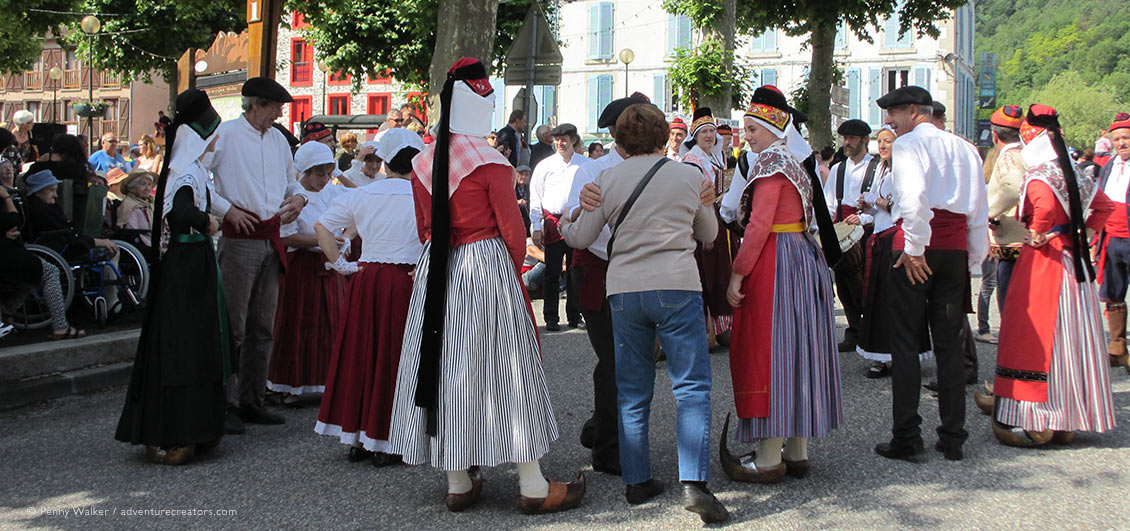In this outdoor photograph, a large group of people is arranged in a big circle, suggestive of an imminent dance performance. They are dressed in traditional Dutch attire, signaling a festival or celebration, possibly in a village reminiscent of the Netherlands, as indicated by the white stucco buildings with brightly colored window frames and shutters in the background. The men wear white shirts, black pants, black beret caps, and wide red sashes around their waists. The women, dressed in old-fashioned Dutch costumes, sport long skirts with vertical stripes in dark green and dark red, complemented by thick cloth hose and wooden clogs with pointed, upturned toes. Their outfits are completed with red aprons, red long-sleeve tops, and yellow belts around their waists. Each woman also wears a shawl-like headdress that covers their hair and drapes over their shoulders, hanging down pointedly at the back and front. In the background, spectators, including a woman in a wheelchair with a blue hat and other onlookers, are visible. A woman in blue jeans, a sweater, with a purse, and black shoes stands near the crowd, emphasizing the gathering's vibrant and inclusive atmosphere.